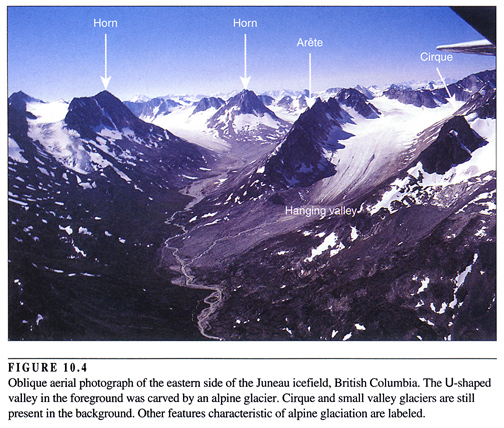The photograph depicts a dramatic landscape of the eastern side of the Juneau Ice Field in British Columbia, captured from an airplane, evident by the visible tail fin in the upper right corner. Dominating the scene are multiple black, jagged mountain peaks covered with snow and ice fields just below their summits, against a striking blue sky. Prominent features of alpine glaciation are highlighted with white arrows and labeled in white text. On the leftmost peak, an arrow points to it indicating it is a "horn." In the central part of the image, another black peak is similarly labeled as a "horn," and further to the right, arrows identify an "arête" and "cirque." Below, a wide U-shaped valley carved by an alpine glacier extends into the forefront, with a "hanging valley" label positioned centrally. The bottom of the image contains a descriptive caption in black text on a white background reading: "Figure 10.4: Oblique aerial photograph of the eastern side of the Juneau Ice Field, British Columbia. The U-shaped valley in the foreground was carved by an alpine glacier. Cirque and small valley glaciers are still present in the background. Other features characteristic of alpine glaciation are labeled." The photograph interweaves the stark contrast of the black peaks with the pristine white snow, capturing a breathtaking example of glacial terrain.